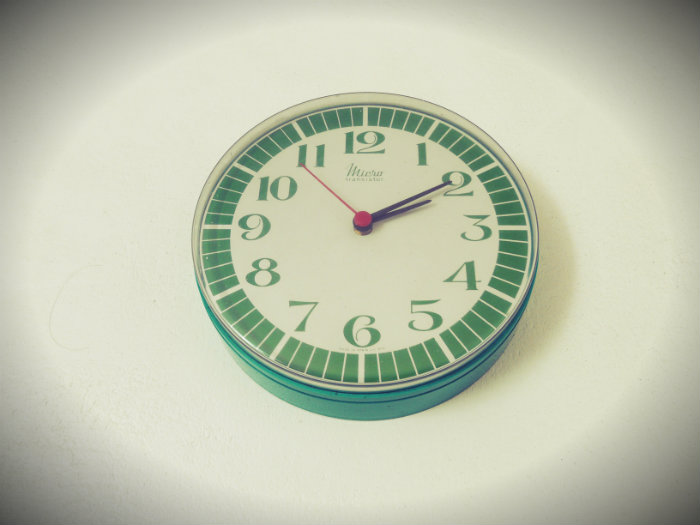This image captures a clock characterized by vibrant green numbers and encased in a green frame, which appears to be crafted from either metal or plastic. Surrounding the clock face, there is a series of short lines forming a border around the numbers, adding a decorative element. The clock features three hands: a large minute hand and a small hour hand, both pointing towards the two, and a red second hand nearing the eleven. The overall design is both functional and visually appealing, with the green elements providing a striking contrast against the more subtle frame.